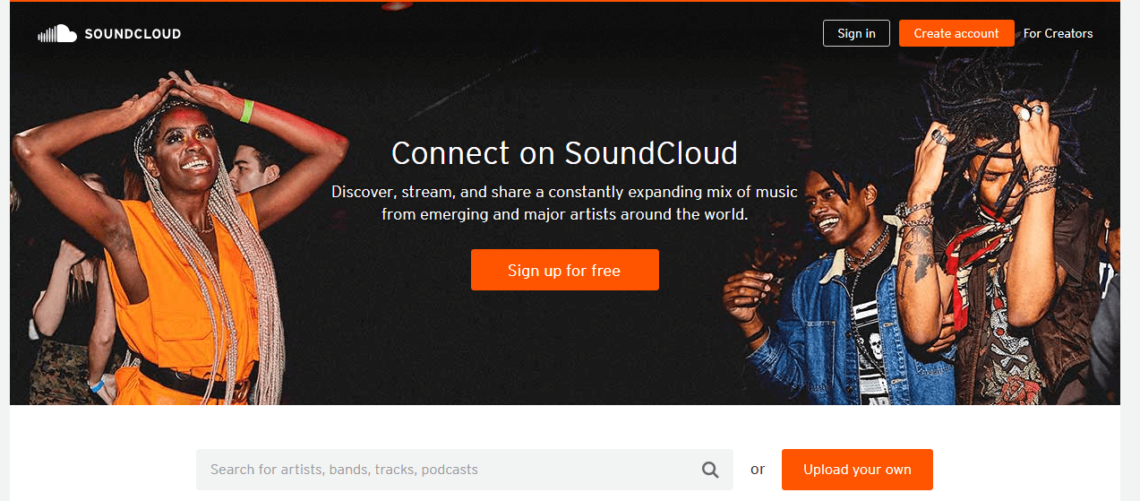This image, sourced from the SoundCloud website, features a vibrant and engaging layout that emphasizes user interaction and creativity. In the upper left corner, the SoundCloud logo is prominently displayed, depicting a cloud with distinctive white lines streaming down from one half and a solid white fill on the other. 

Across the top of the webpage, there's a black rectangular sign-in button outlined in white. Next to it, an orange button labeled "Create Account" is easily noticeable, accompanied by a subtle text link for creators. 

Central to the page is a welcoming message: "Connect on SoundCloud," encouraging users to "Discover, stream, and share a constantly expanding mix of music from emerging and major artists around the world." Below this message, an orange button invites users to "Sign Up for Free."

The image showcases a lively scene with several individuals dancing. On the left, an African-American woman with long, blonde braids, dressed in an orange shirt, joyfully raises her hands above her head while smiling broadly. To the right, two African-American men, both with brown hair—one sporting braids or dreadlocks—are energetically dancing. 

Towards the bottom of the page, another orange button appears, offering the options "Sign up for free" or "Upload Your Own" music, encouraging users to engage and contribute to the platform.